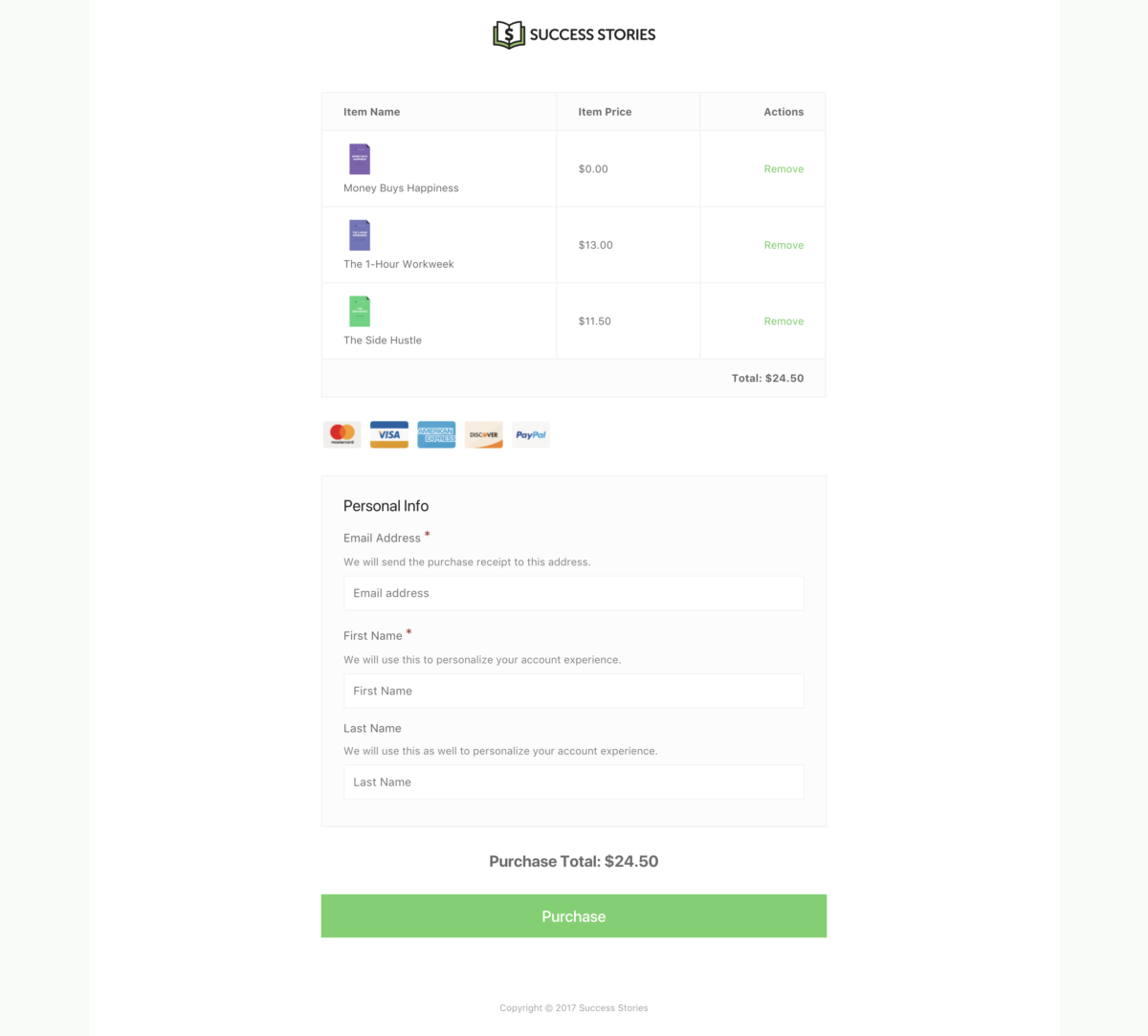The image depicts an eBook checkout page from an online store named "Success Stories." At the top of the page, there is a distinctive icon of an open book with a dollar sign in the center. Right next to it, in large black letters, the store's name "Success Stories" is prominently displayed.

The main section of the page is divided into three columns: Item Name, Item Price, and Actions. Listed under Item Name, the eBooks are titled "Money Buys Happiness," "The One Hour Work Week," and "The Side Hustle." Corresponding to these titles, the Item Prices are $0, $13, and $11.50, respectively. The Actions column features a "Remove" option in green for each item. Summing up the item prices, the Total at the bottom right of this section is $24.50.

Below the itemized list, the Payment Options section is centrally positioned and displays various icons for payment methods including MasterCard, Visa, American Express, Discover, and PayPal.

Further down, the Personal Information section is identified by the bold title "Personal Info." Here, fields are provided for the user to enter their "Email Address," "First Name," and "Last Name." Each field is accompanied by a brief note indicating its purpose: the email address will receive the purchase receipt, while the first and last names will be used to personalize the account experience. Currently, all the fields are blank.

At the bottom of the page, the Purchase Total is reiterated in black text as $24.50. Immediately below this is a prominent lime green "Purchase" button, intended to complete the transaction.